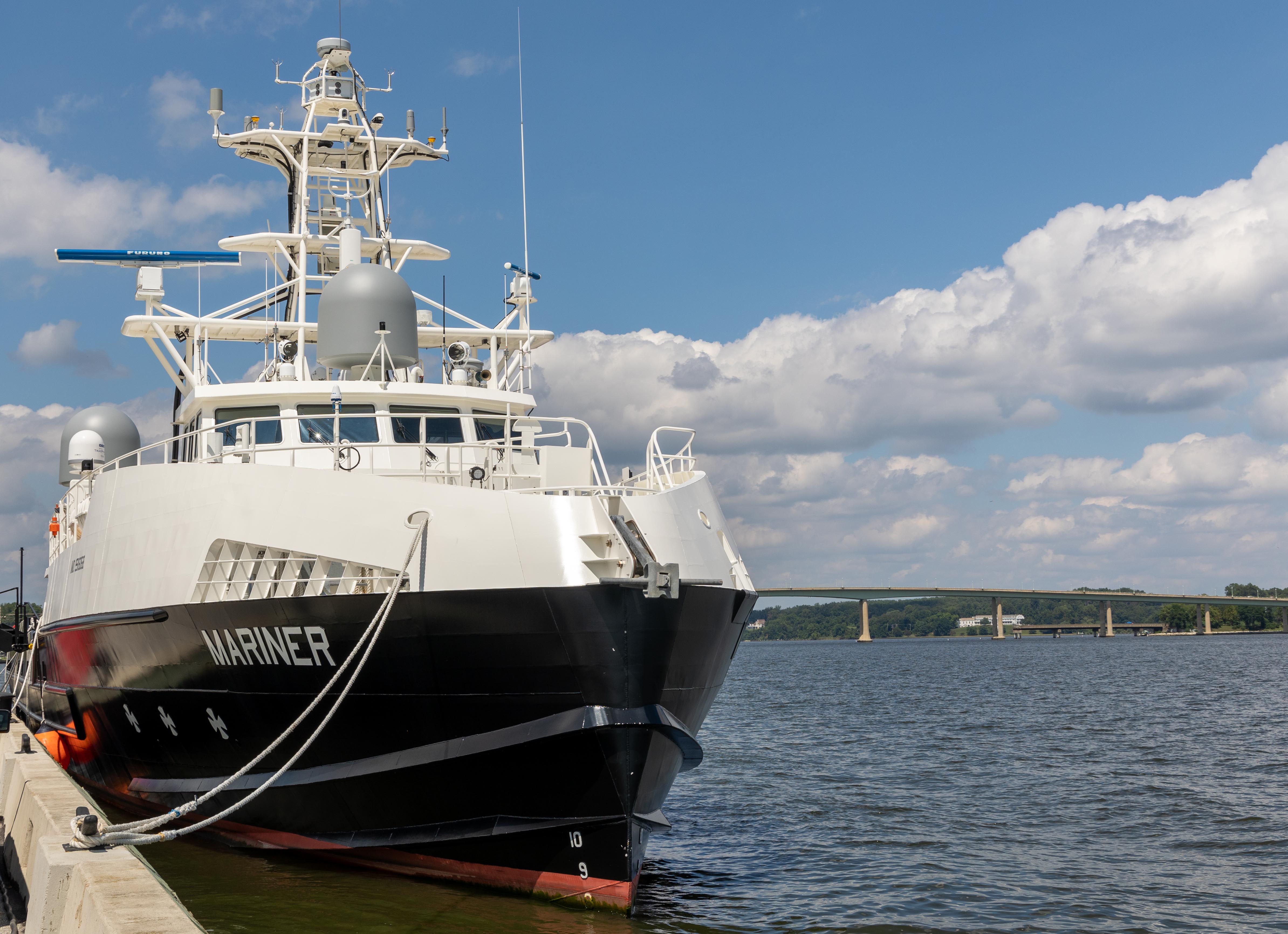In this bright and detailed photograph, a large boat named "Mariner" is prominently docked to the left. The vessel features a black or navy blue hull and a white upper section. Its structure includes various white components, a glass-encased cabin, and a communications tower with what appears to be a ladder on top. Around the boat, ropes are visibly tied to anchors on a concrete dock. Above, the sky is a vivid blue, scattered with large, fluffy white clouds that have hints of gray. The calm, blue ocean water mirrors the peaceful ambience of the scene. In the background, a long bridge stretches across the water, with trees and a large white house visible in the distance. This vessel, more substantial than a pleasure yacht, suggests it serves commercial purposes.